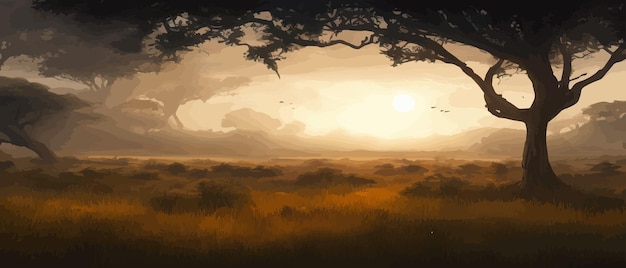The image is a dramatic, wide, color illustration of an expansive landscape, possibly set in Africa, showcasing a vivid sunset or sunrise. The scene is dominated by a large, shadowed tree with a broad canopy on the right side, while another similarly large tree is positioned in the middle ground on the left. The field below is illuminated in a golden light, highlighting brown, leafy grasses and vegetation. Scattered throughout the background are several smaller trees, creating a sense of depth. The horizon features a brilliant yellow sun that radiates light across the landscape, casting dynamic shadows and lending a warm glow to the scene. Above, a clouded sky hosts silhouettes of six birds in flight, some distinctly visible and others partially obscured by the tree branches. The entire scene, rich in detail and color, appears to be a computer-generated illustration, capturing the essence of a serene yet dramatic landscape.